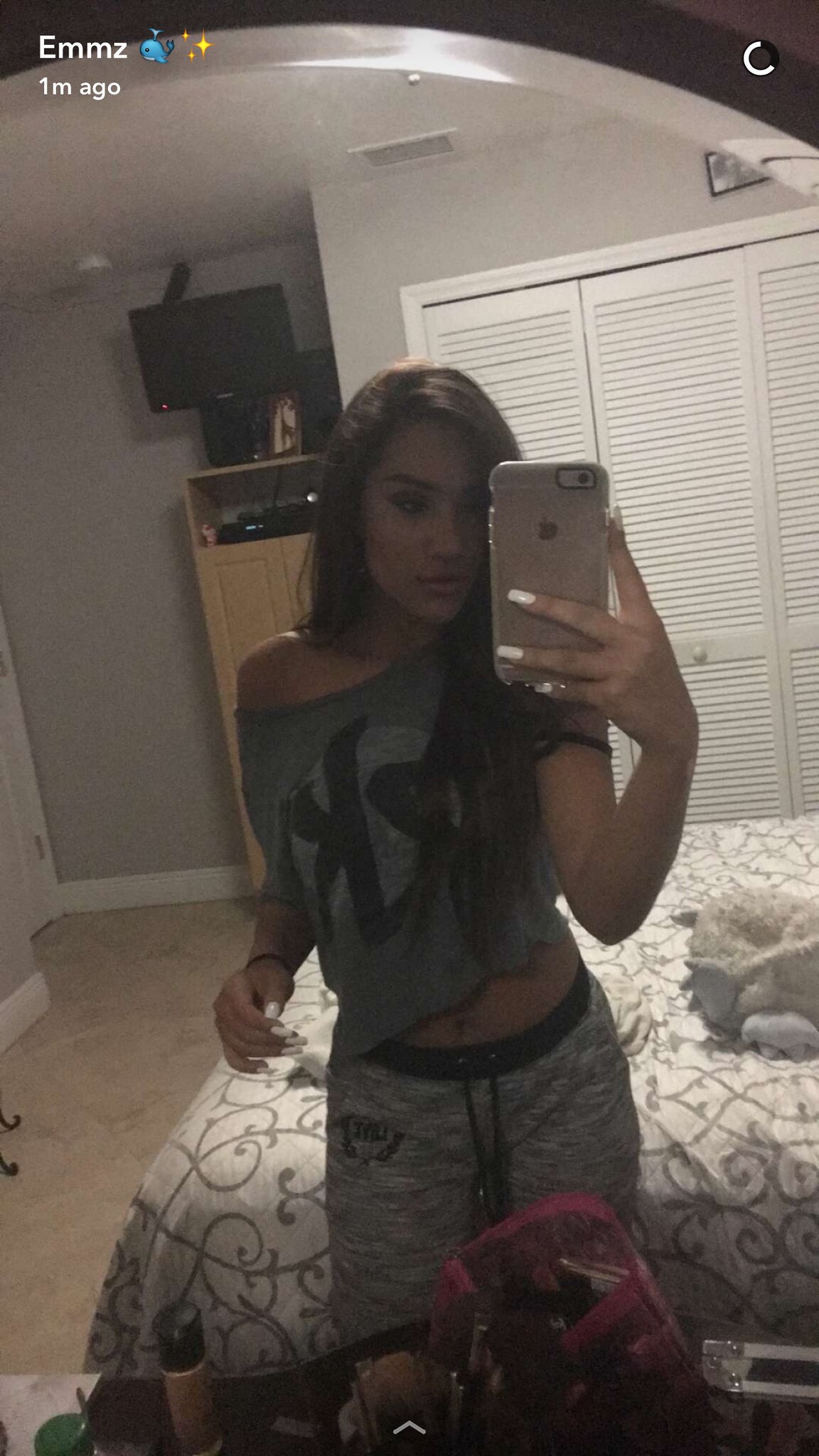This detailed photograph captures a young woman taking a selfie in her bedroom, likely intended for social media. The image shows her standing in front of a round mirror, holding a silver iPhone with a whale emoji and a magic star emoji next to her username 'Ems' (E-M-M-Z), indicating the photo was posted one minute ago. She has long brunette hair and is wearing gray pajama pants with a black waistband, paired with a loose-fitting crop top that hangs off one shoulder. Her long white nails are clearly visible as she extends her arm to take the picture. Her room is decorated with gray walls and white closet doors, and contains a TV mounted close to the door, a bed with a white blanket, and a desk with various makeup items. The floor appears to be carpeted in tan, and the overall setting is well-lit, showcasing a cozy and personal space.